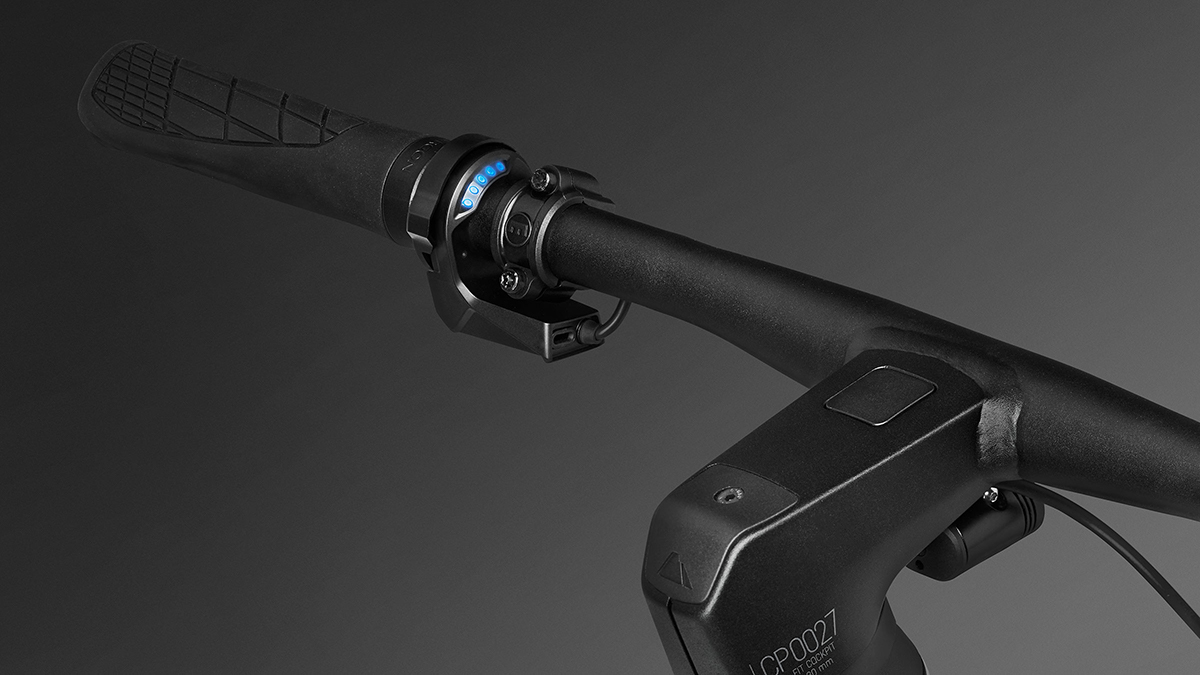This is a close-up photograph of what appears to be the left handlebar of a stationary or exercise bike. The handlebar is predominantly black, constructed from metal, and features a black leather grip adorned with a possible brake lever or adjustment dial. The handlebar has a premium, matte black finish and includes a wired connection that likely tracks workout progress or connects to a smart device for monitoring. The background displays a gradient from black in the upper left to dark gray in the lower right, enhancing the sleek, modern look of the handlebars. Visible on the metal bar is a partially cut-off engraving, showing "CP0027." The image focuses solely on the left handlebar, providing a detailed and close-up view while leaving the right side out of frame.